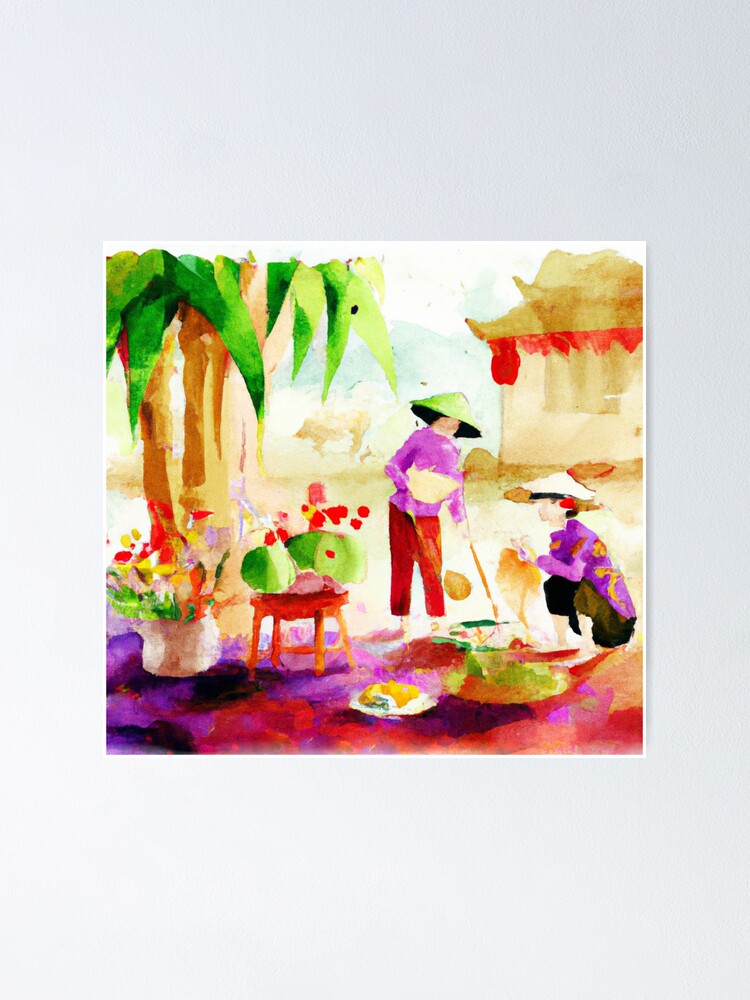The image is a detailed illustration of two women engaged in an outdoor activity, set in what appears to be a Southeast Asian or East Asian environment. Both women are donning traditional conical hats with pointed tops and wearing purple shirts with distinct yellow designs. The woman on the left wears red pants and is standing, holding and pointing at something on the ground with a stool and a pot of vibrant flowers next to her. The woman on the right, dressed in dark pants, is kneeling and appears to be involved in the same activity. The background features a hut or a structure with a thatched roof and palm trees, and the scene is set under a blue sky with hints of red-trimmed buildings. The ground is splashed with purplish-red hues, suggesting a watercolor effect, and there are signs of outdoor cooking, including food spread out on a mat and possibly a pot. The setting also contains a lush green fruit stand and the overall composition evokes the lively and colorful atmosphere of an outdoor scene in Southeast Asia.